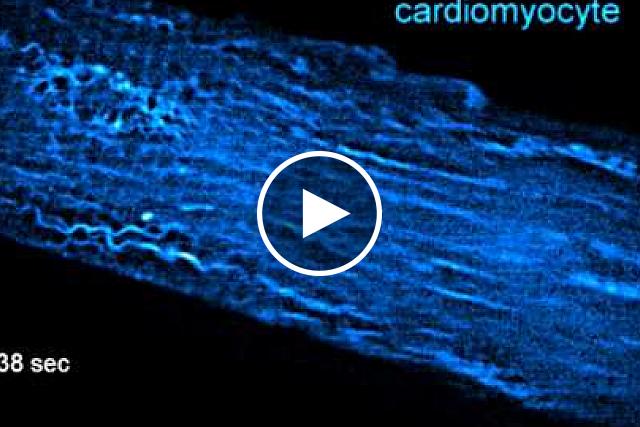This image is a screenshot of a YouTube-like video before it begins playing, featuring a central white play button with a partially transparent triangle and circle design. At the upper right corner, the word "Cardiomyocyte" is displayed in blue text, while the lower left corner shows a white timestamp reading "38 seconds." The background is predominantly black, with a broad blue filament—possibly muscle cells—stretching diagonally from the top left to the bottom right of the image. This filament exhibits striations and various lines, resembling material viewed under an electron microscope, emphasizing the scientific context of the scene. The blue filament appears textured, with smoother and rougher edges indicating folds and ruffles.